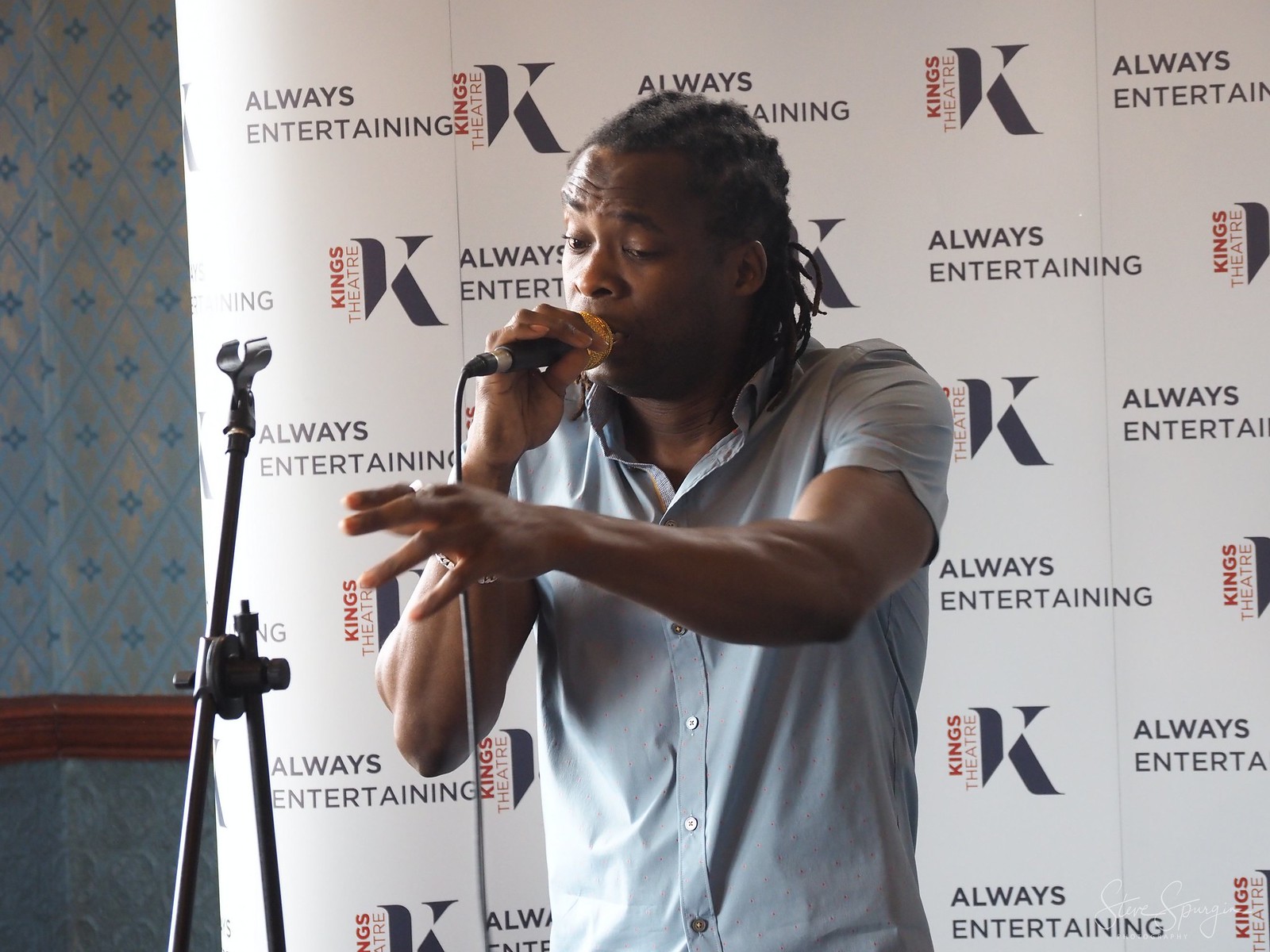The image captures an African-American man, likely in his early to mid-30s, standing on a small stage. He has black dreadlocks or braids and is wearing a light blue, short-sleeve, button-down collared shirt. The man is holding a microphone up to his mouth with one hand, while his other arm is extended, suggesting he's either singing or delivering a speech or comic performance. He stands in front of a backdrop featuring a repeating pattern of signage that reads "Always Entertaining King's Theatre" along with a large, distinctive black "K" logo. The wall behind him also displays a blue and yellow diamond-shaped patterned wallpaper with wood-colored molding running halfway down. The microphone stand is positioned just in front of him, slightly to his left.